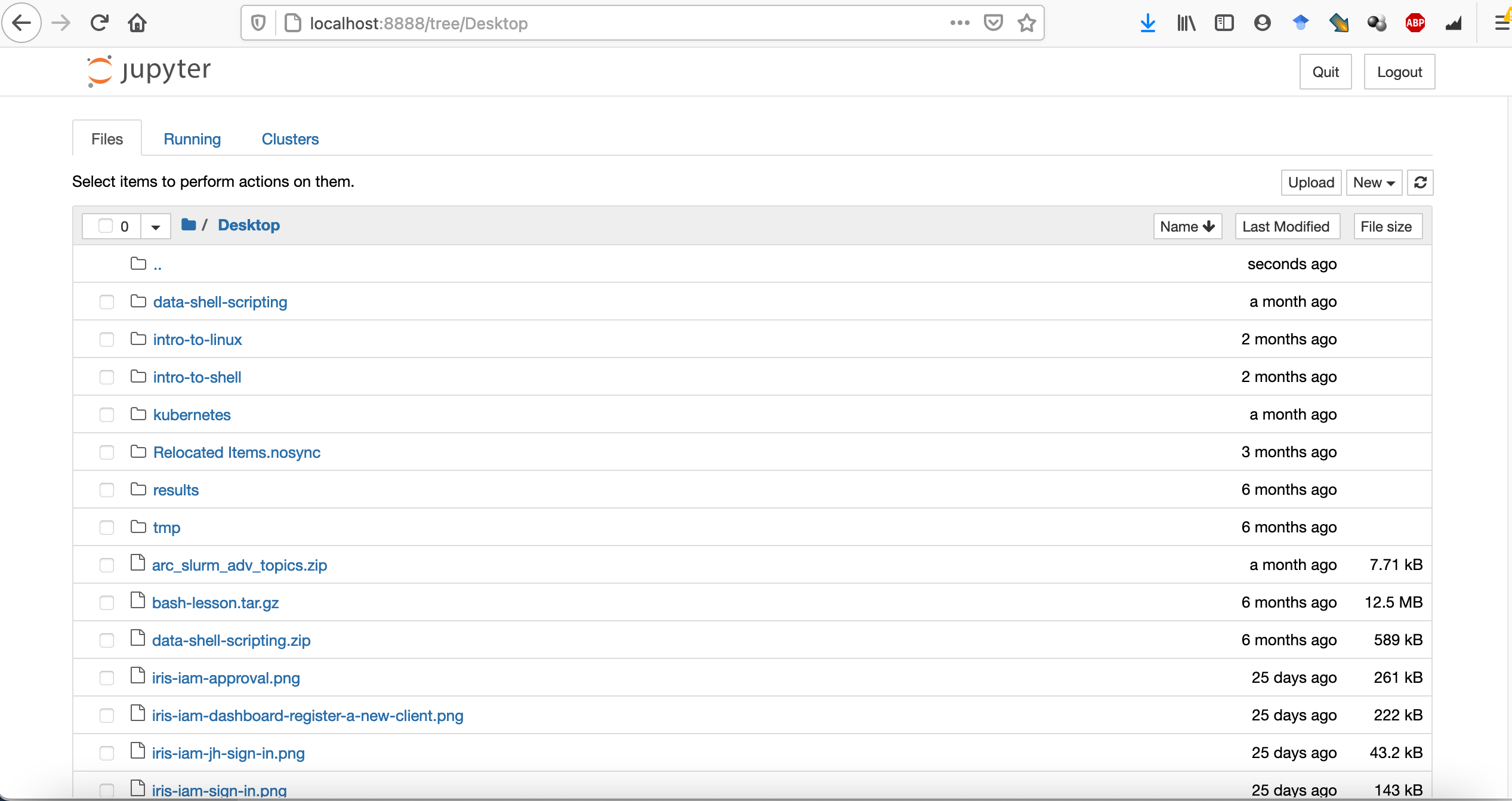This image is a detailed screenshot of a Jupyter Notebook interface running locally on a computer. The browser's address bar shows "localhost" followed by the port number '8888' and the URL path '/tree/desktop'. The word "Jupyter," spelled as "j-u-p-y-t-e-r," is prominently displayed beneath this URL.

The interface is divided into three main tabs situated at the top: 'Files', 'Running', and 'Clusters'. The 'Files' tab is currently active, highlighting a list of various folders and files in a structured column on the left side. Adjacent to each file and folder name are details specifying the "Last Modified" timestamp, which ranges from a few seconds ago to several months ago.

On the far right, file sizes are displayed, particularly for ZIP files, PNG files, and specific documents, whereas directory folders do not show an aggregated size. This meticulous organization aids in easy navigation and management of various files and resources within the Jupyter Notebook environment.